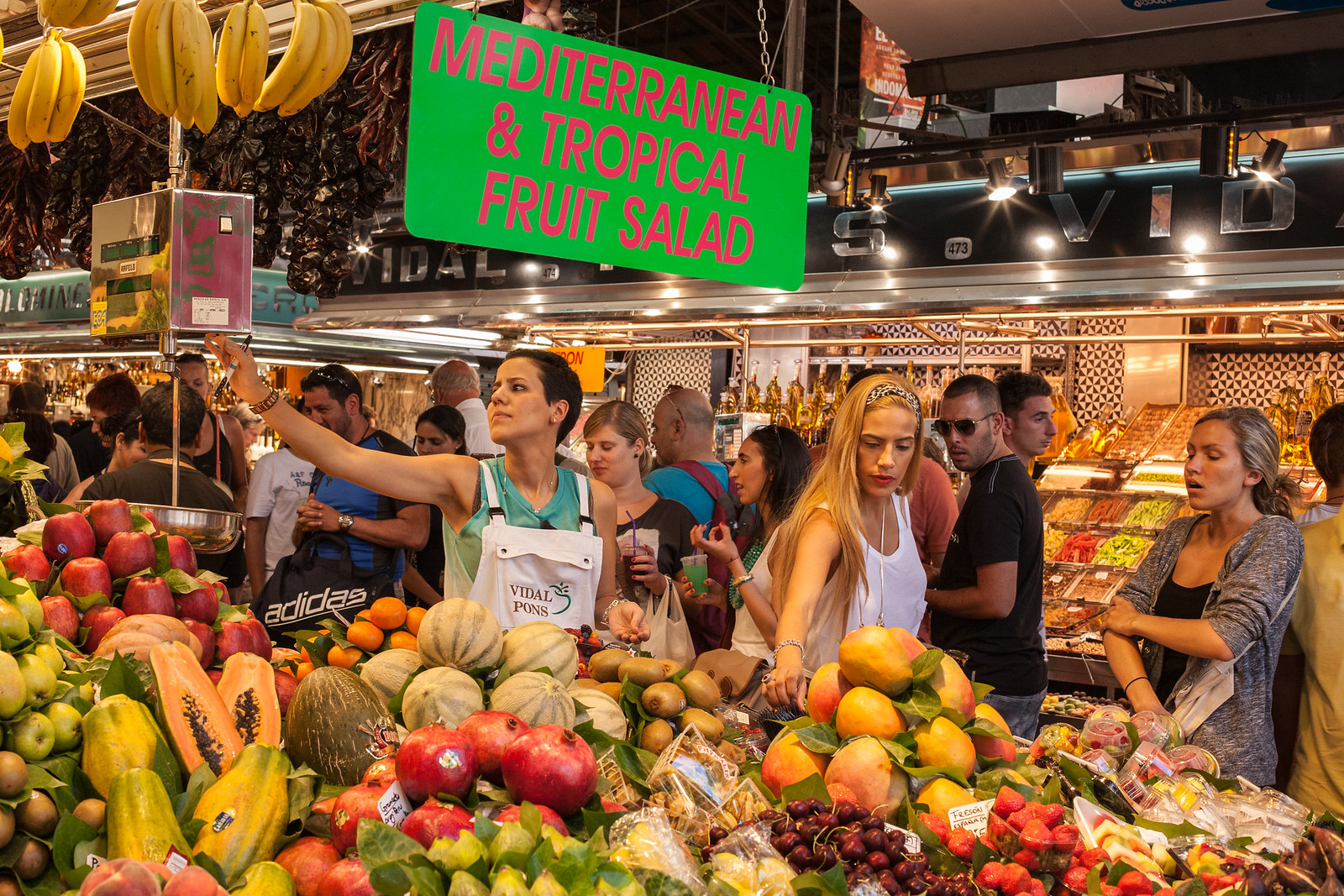This vibrant, full-color photograph captures a bustling farmer's market scene, brimming with an array of fresh produce and active shoppers. The market setting appears to be a large open area, possibly indoor given the overhanging metal rods and what seems to be storage trunks overhead. A prominent green sign with bold, red, right-slanted text announces "Mediterranean and Tropical Fruit Salad."

In the foreground, the market stand overflows with a colorful assortment of fruits. There are bunches of bananas hanging from the metal rods, alongside a variety of other tropical fruits including pomegranates, berries, kiwi, melons, strawberries, and grapes. Some melons are sliced open, adding to the visual feast. To the left, a woman in white overalls and a green sleeveless top extends her arm toward the hanging bananas, seemingly in charge of the stand. She wears an apron, suggesting she's a vendor.

Nearby, a tall blonde woman with flowing hair and a white tank top reaches for a piece of produce near a pile of papayas. Another woman, slightly older, dons a black top with a sweater jacket and stands with her arms semi-folded, contemplating the fruit selection without touching it. The market is lively with shoppers, including a few more individuals moving in different directions—among them a man glancing toward the blonde woman and a dark-haired woman passing by her.

In the background, additional rows of fruits and packaged items suggest a well-stocked and diverse market, promising a rich shopping experience for its patrons.